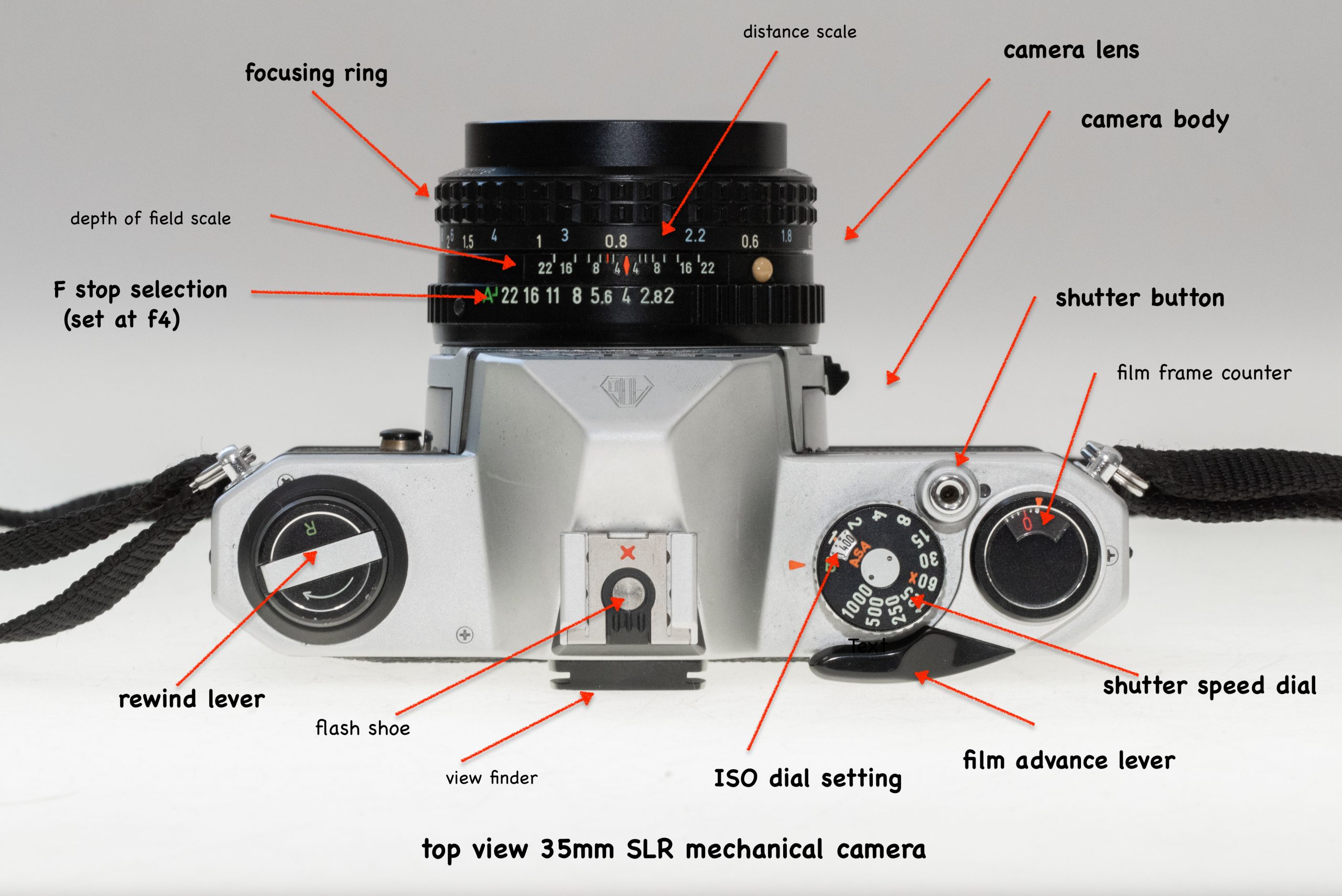This is a detailed infographic showing the top view of a 35mm SLR mechanical film camera. The camera is silver with a black lens featuring numbers and letters for aperture settings, currently set at f4. It is laid on its back with the lens pointing upwards. Various red arrows point to different components, each labeled with black text identifying the parts.

Starting at the top and moving clockwise, the labels include:

- **Distance Scale**: This points to the top row of numbers on the camera lens.
- **Camera Lens**: The central black lens with specified numbers for aperture values. 
- **Camera Body**: The main silver structure of the camera.
- **Shutter Button**: Located near the center, used to take pictures.
- **Film Frame Counter**: Displays the number of frames used.
- **Shutter Speed Dial**: A circular dial to adjust the shutter speed.
- **Film Advance Lever**: Found on the left side, used to advance the film after taking a photo.
- **ISO Dial Settings**: For adjusting the camera's sensitivity to light.
- **Viewfinder**: The black part you look through, situated near the top center.
- **Flash Shoe**: Positioned above the viewfinder for attaching an external flash.
- **Rewind Lever**: Located on the left side for rewinding the film.
- **F-stop Selection**: Dial set at f4 to control the aperture.
- **Depth of Field Scale**: Shows the range of sharp focus.
- **Focusing Ring**: Surrounds the lens for adjusting focus.

The camera also features black neck straps attached to either side. Black text at the bottom of the infographic identifies it as a "Top View of a 35mm SLR Mechanical Camera."